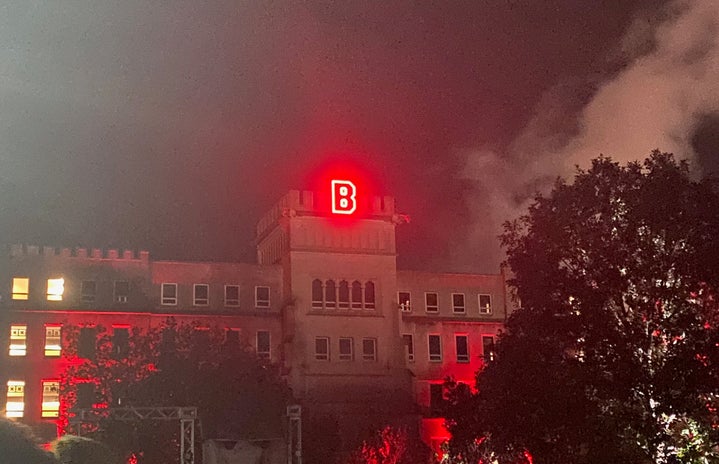A large, light-colored building with at least three floors stands against a dark night sky, characterized by its plain and slightly dated architecture. In the center of the building, a white neon capital "B" glows brightly at the top of a slightly taller section. Rows of tall, rectangular windows align each floor, with the ones in the center appearing blacked out. On the left side of the image, six windows are lit up from the inside, arranged in two vertical columns of three. A fog or smoke envelops the right side of the building and spreads into the sky, adding an eerie atmosphere. In front and overhead of the building, trees obscure parts of the facade, with faint light shining through their branches on the right side.